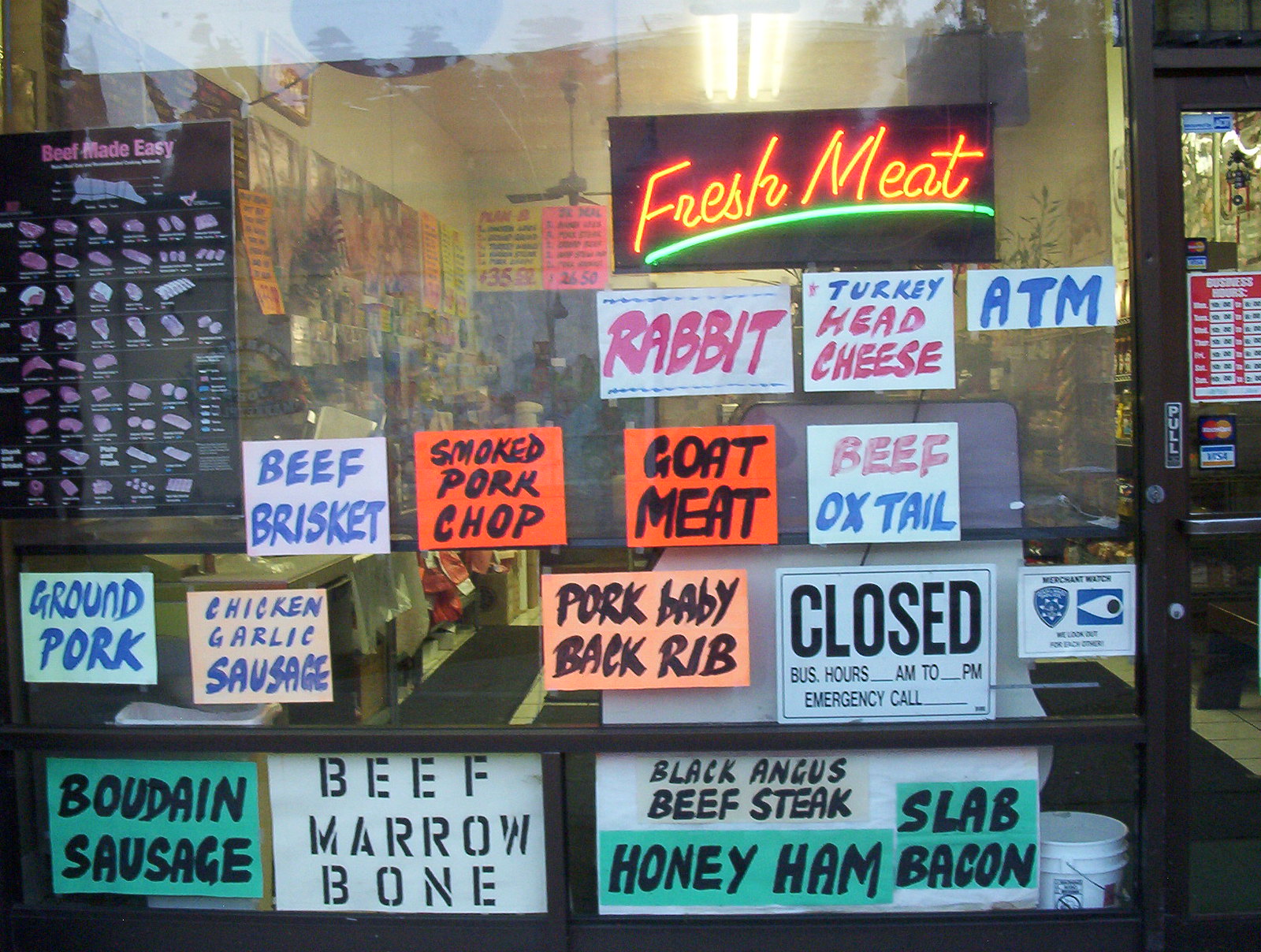The photograph showcases the front of a meat market or restaurant, centered on a large, transparent glass window adorned with numerous posters and handwritten signs, detailing an extensive menu. Prominently displayed is a lit sign in yellow and green lights stating "Fresh Meat." Surrounding this sign, among various colored papers, are specific items including rabbit, goat meat, beef brisket, smoked pork chop, turkey head cheese, ATM, beef oxtail, ground pork, chicken, garlic sausage, pork baby back ribs, boudin sausage, beef marrow bone, black Angus beef steak, honey ham, and slab bacon. The posters are arranged in clusters, with a series of smaller white and orange signs below the main text segments. The lower part of the window features more signs and a closed sign in bold black letters. A brown border runs along the bottom of the window, above which is a white bucket in the bottom right-hand corner. To the right of this expansive window is a glass door marked with a plaque that reads "Pull," and store hours are indicated on an upper window panel of the door. The setting is outdoors in daylight, with a visible glimpse inside the shop through the transparent glass. Various colors dominate the scene, including pink, black, gray, light blue, dark blue, teal, orange, green, and tan, enriching the vibrant yet bustling atmosphere of the storefront.